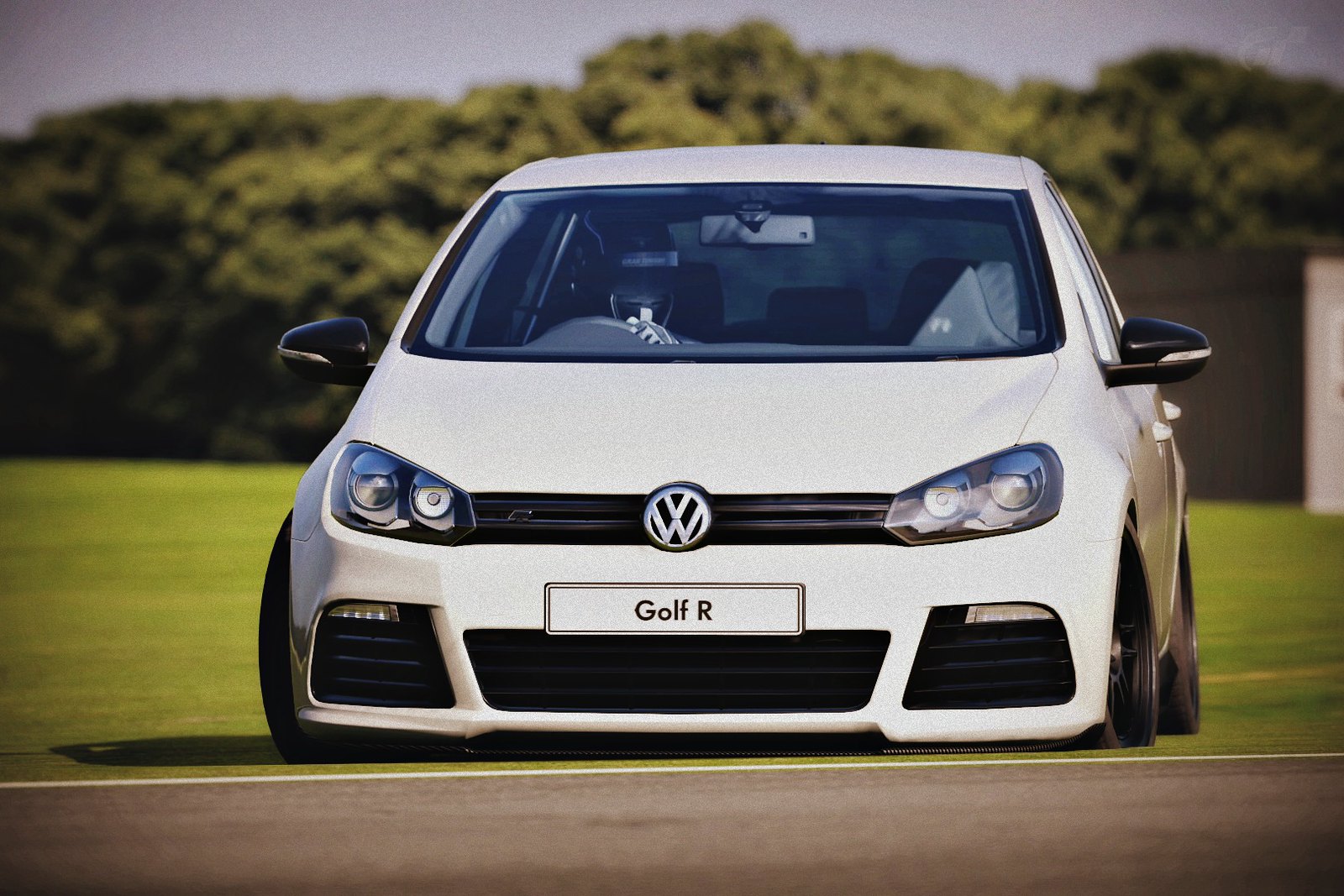The photograph captures a pristine, white Volkswagen Golf R parked on well-manicured grass, with a clear blue sky overhead. The front-facing car prominently displays the VW logo and a nameplate reading "Golf R" where the license plate would typically be. The vehicle features black accents, including the grille and side mirror holders, which also have integrated blinkers. The driver, wearing gloves and a helmet suggestive of a race car driver, is seated in the black interior, gripping the steering wheel. The background showcases a lush, green landscape with slightly out-of-focus trees, indicating a sunny and cloudless day. Additionally, there is a strip of asphalt visible in the foreground, leading up to the car.